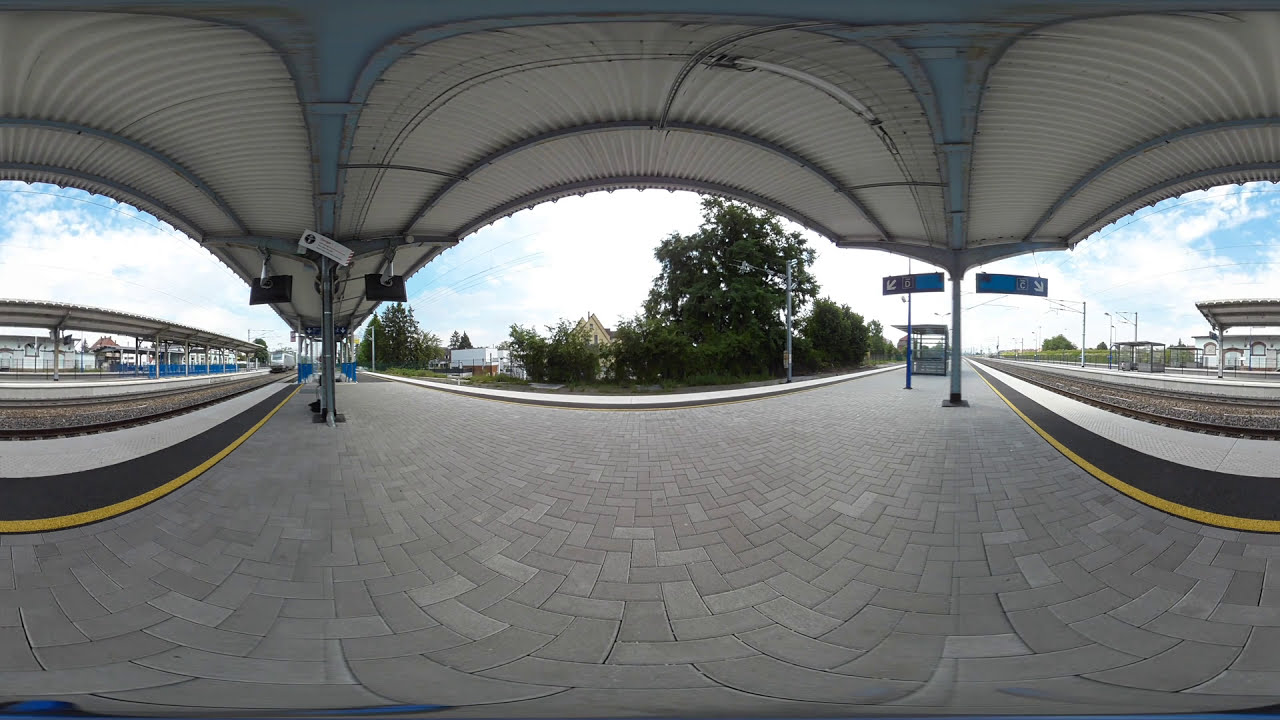The image is a 360-degree panoramic view of a light rail station platform. The platform is paved with gray bricks and features two curved walkways extending away from the viewer. There are railway tracks on both the far right and left sides of the image. On the right side, the track is bordered by a white strip followed by a black strip with yellow guidelines. Overhead, a metal structure supports a roof, likely made of a material similar to hard plexiglass or sheet metal, providing shelter for waiting passengers. This metal frame with white roofing appears consistent throughout both sides of the image.

On the far right, there is a station with signboards mounted on two pillars, and across the train track, another shed similar to the one in the foreground is visible, along with a white building behind it. The left side mirrors this setup, with another shed and metal frame parallel to the tracks.

Surrounding the platform are trees, some pine, and bushes. The distant background showcases a sidewalk curving around the vegetation and some indistinct buildings, possibly houses, under a blue sky filled with clouds. Light posts dot the landscape, enhancing the station's ambiance. The panoramic distortion emphasizes both the gray brick ground and the metal awning overhead.